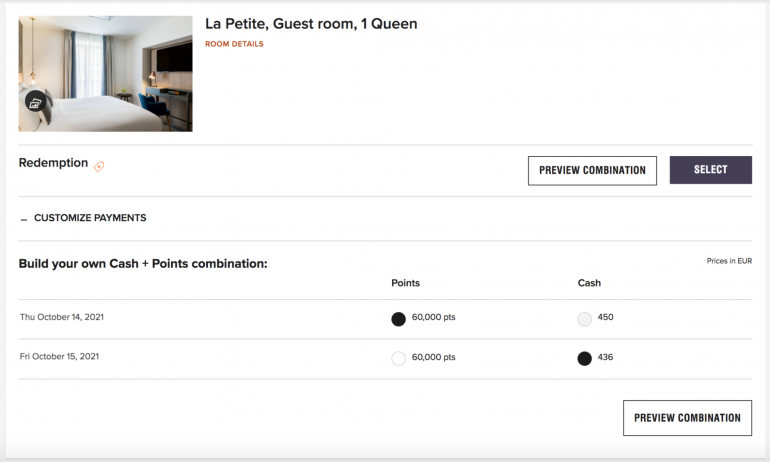This image depicts a sleek webpage interface for confirming a hotel reservation at La Petite Guest Room. The layout is landscape-oriented, approximately twice as wide as it is tall, encapsulated within a gray border and set against a white background.

In the upper left corner, there is a photograph of the hotel room, showcasing a typical setup of a bed on the left and a TV on the right. Adjacent to this image, in bold black text, is the room description: "La Petite Guest Room One Queen." Below the room description, the phrase "room details" is highlighted in a brownish-orange hue.

A horizontal gray line delineates this section from the next. The new section starts with the word "redemption" in black, bolded text on the left, accompanied by a small orange ticket icon aligned to its right. Further to the right, there are two interactive buttons: a white button outlined in black with the text "preview combination," and a black button with white text labeled "select."

Another horizontal gray line separates this from the subsequent section titled "customize payments." Continuing downward, yet another horizontal gray line introduces the final section, prominently stating "build your own cash plus points combination" in bold text.